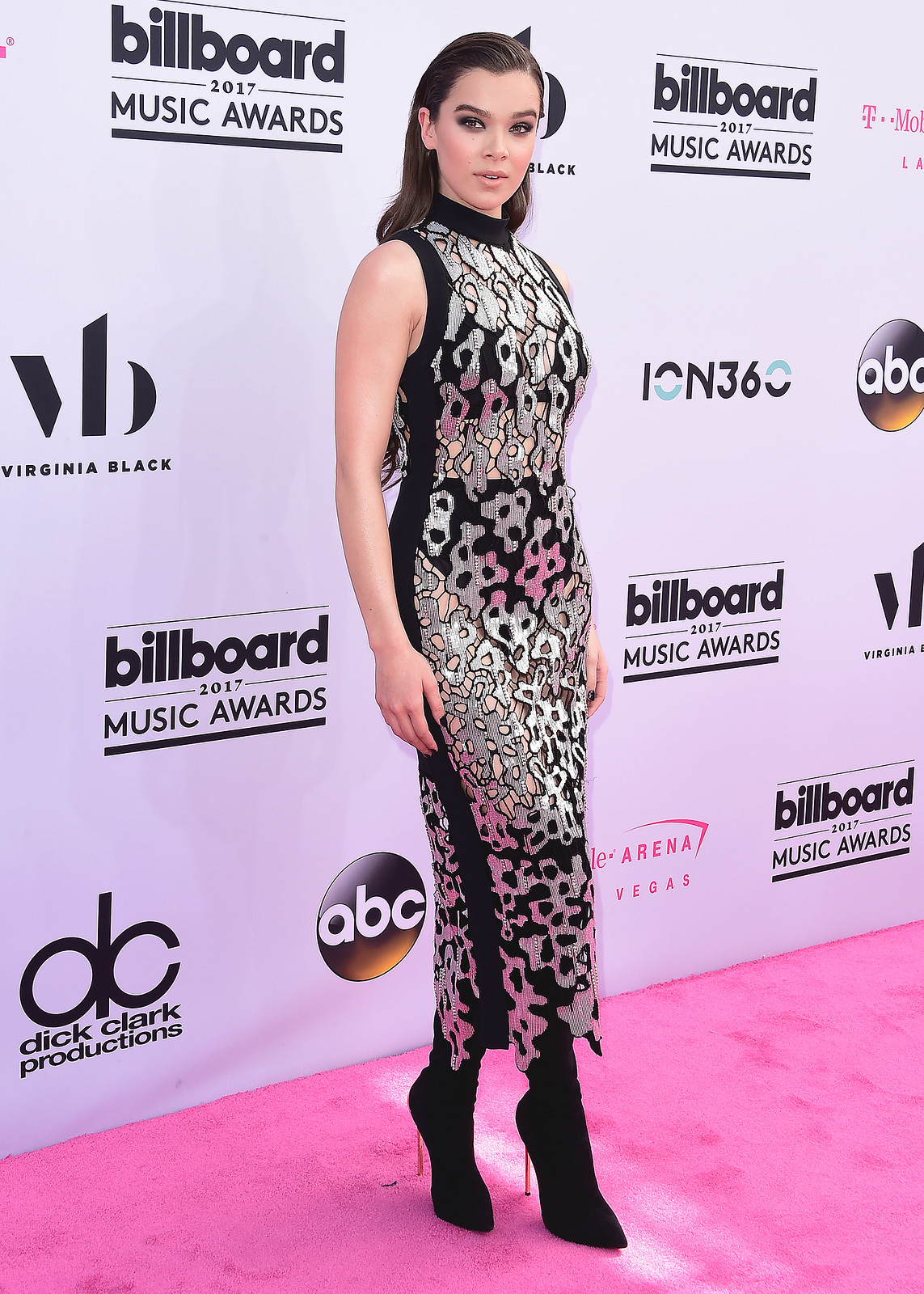This photograph captures a woman attending the Billboard Music Awards 2017, posing on a pink carpet in front of a white backdrop adorned with logos for Billboard Music Awards 2017, ABC, and Dick Clark Productions. The woman has long brunette hair slicked back, and dark eyes, accentuating her sophisticated look. She is dressed in a striking, see-through long dress that reaches her ankles, featuring a black background with a silver animal print, and complemented by black high-heeled boots. The sleek design of her outfit reveals a black bra and black underwear underneath. She gazes directly into the camera, exuding confidence and elegance.